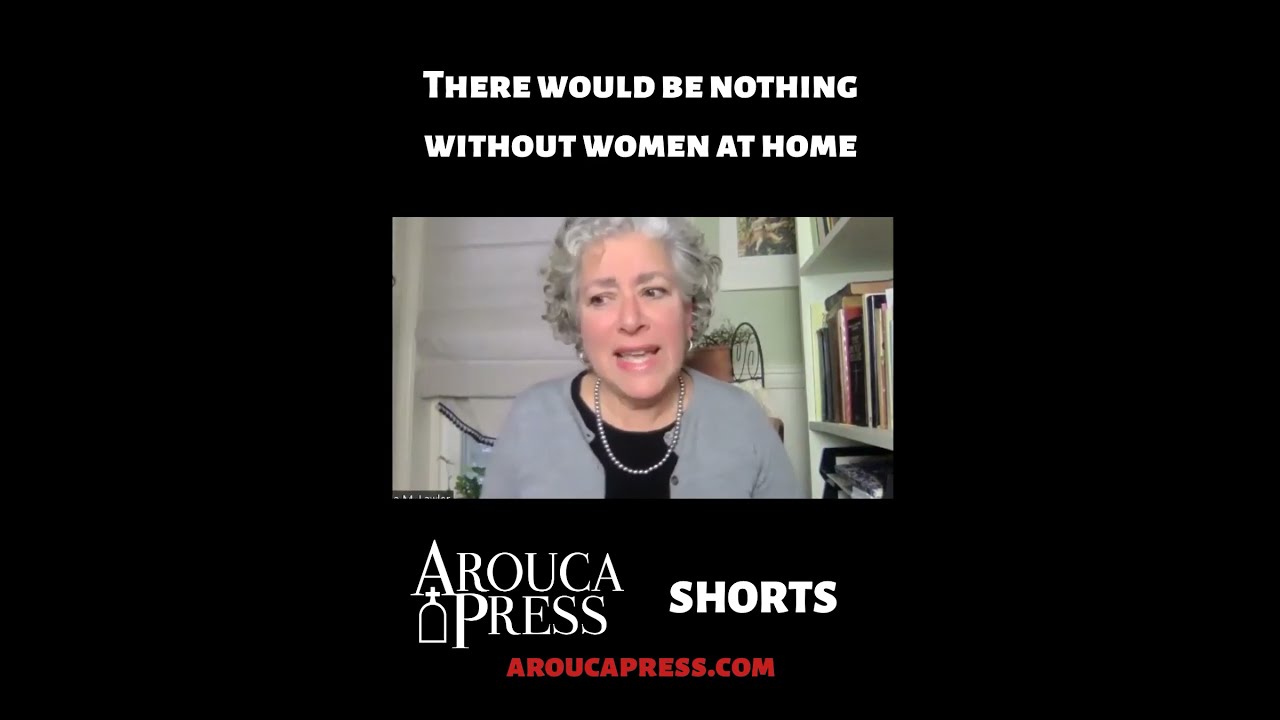The photograph portrays an older woman with short gray hair, dressed in a gray cardigan sweater over a black top, complemented by a pearl necklace. She appears to be speaking while facing the camera. The background of the image is black, with additional black strips on the sides, creating a central framing for the photo. Behind the woman, there's a window with a gray shade, a bedroom setting, and a shelf with several books on the right side. The room also features pictures on the wall and possibly a plant. Above the image, in white text, it reads, "There would be nothing without women at home." Below the image, additional white text states, "Arouca Press, shorts," followed by the URL "aroucapress.com" in red.